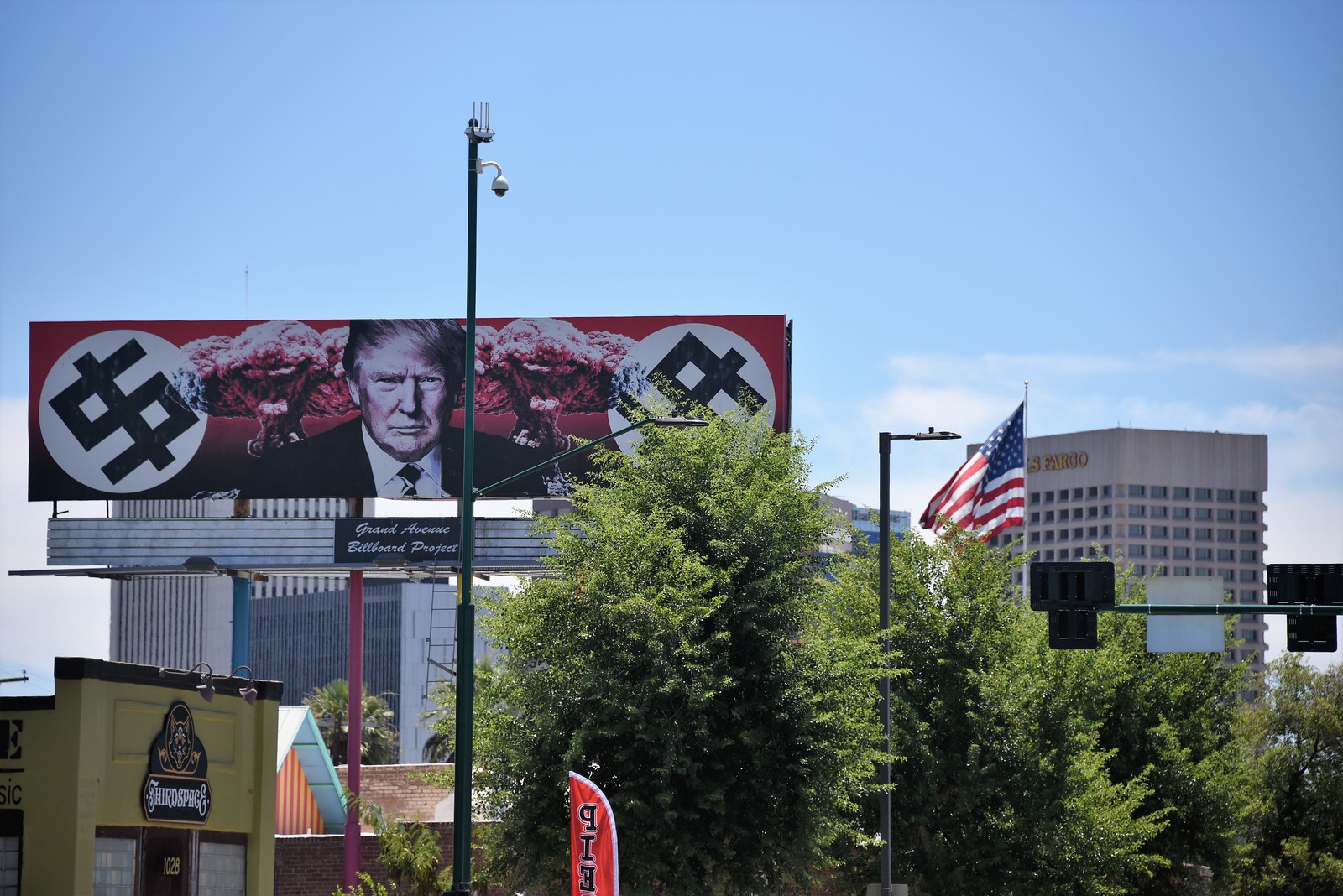The image captures the side of a road with a vivid blue sky adorned by dusty clouds. Prominently positioned is a large billboard with a striking red background. The billboard features an image of Donald Trump donning a black suit, white shirt, and black tie. Flanking him on both sides are two large white circles, each bearing a black symbol that fuses a dollar sign with a Nazi swastika. Behind Trump, dramatic depictions of explosions and puffs of smoke create an intense visual. Below the billboard, there's a glimpse of a yellow building. In the foreground, a red shop flag is visible along with several tall trees, rich with green leaves. An American flag flutters on a gray pole, adding a patriotic touch, while a green telephone pole and a purple pole support the surrounding infrastructure. In the distance, tall buildings rise up, completing the scene with an urban backdrop.